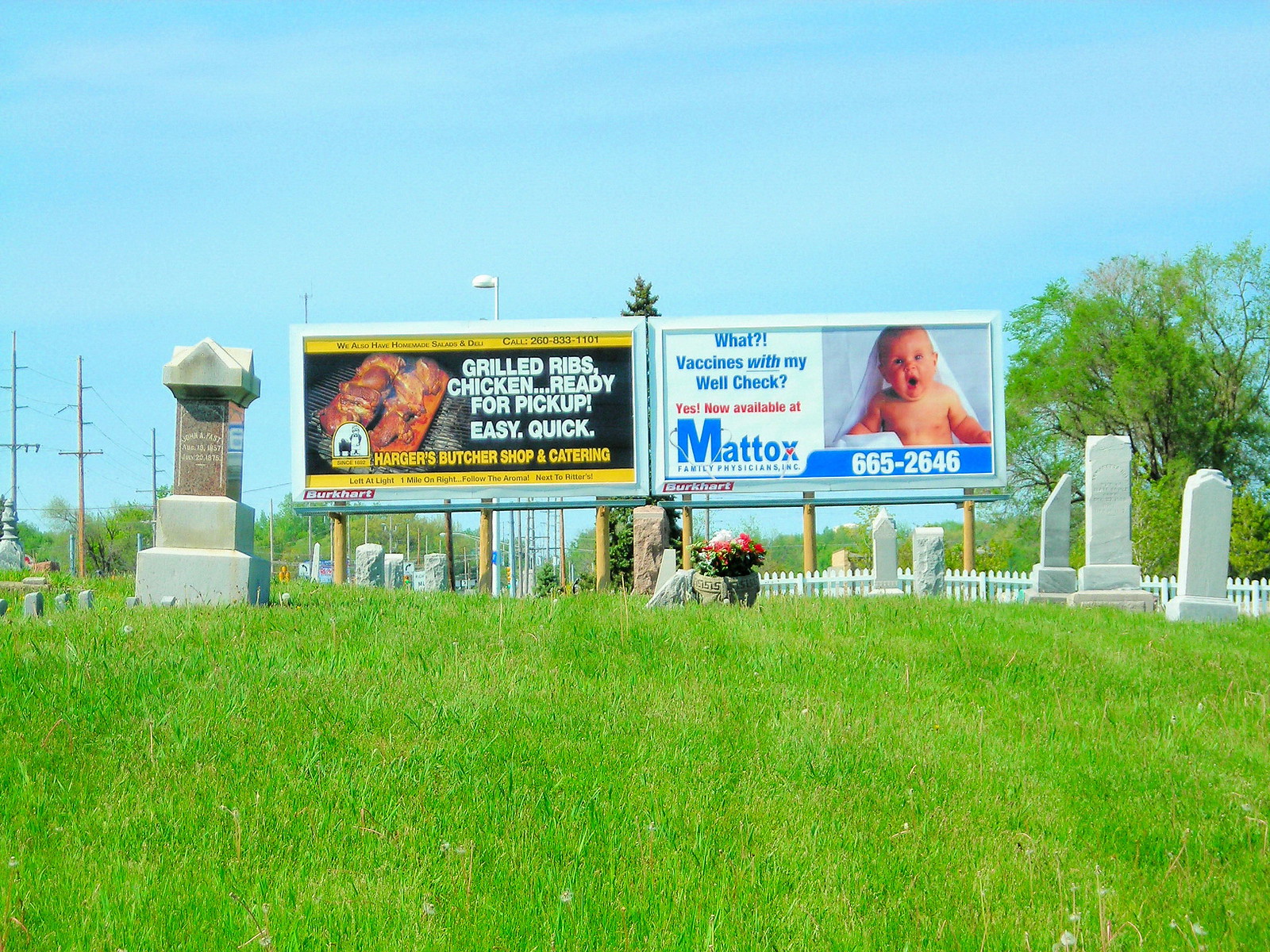On a bright summer's day, the image captures a vibrant scene from the perspective of someone lying on lush, green grass, gazing upward towards a remarkably clear sky. Dominating the center of the background are two large billboards that draw immediate attention. The first billboard advertises Hargers Butcher Shop and Catering with a tempting visual of grilled ribs and chicken. The advertisement, set against a black background with a yellow trim, highlights the ease and convenience of picking up their expertly prepared meats. The second billboard promotes vaccine availability at Matic, featuring an image of a baby alongside text encouraging well-check visits and a contact number for further information.

In the foreground, a graveyard spreads across the grassy expanse, dotted with various gravestones that add a solemn touch to the setting. A small white fence lines one side of the graveyard, accompanied by a scattering of trees that provide a subtle natural border. Additionally, a few telegraph poles are visible to the left, blending into the serene yet slightly bustling landscape.